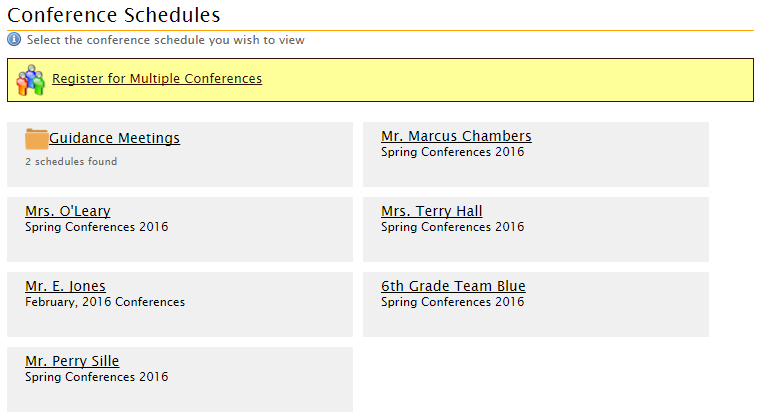The image features a detailed conference schedule layout. At the top of the image, a yellow bar spans across the screen, containing a prominent notification symbolized by an "i" inside a circle, indicating important information. Directly below, it instructs viewers to "Register for multiple conferences" in black text.

Beneath this notice, there is a colorful cartoon image depicting three characters: one in orange, one in blue, and one in green, adding a touch of illustration to the otherwise text-heavy image.

The main section of the image displays a series of conference schedules with associated names and details, each separated by grayish-white boxes. Here are the highlighted schedules:
- Guidance Meetings, indicated by a folder icon next to it, with a note stating "2 schedules found."
- Mr. Marcus Chambers, "Spring Conferences 2016."
- Ms. O'Leary, "Spring Conferences 2016."
- Ms. Terry Hall, "Spring Conferences 2016."
- Mr. E. Jones, "February 2016 Conference."
- 6th Grade Team Blue, "Spring Conferences 2016."
- Mr. Perry Seil, "Spring Conferences 2016."

All names and labels are written in black text, providing a clear and organized visualization of the various conference events and their corresponding hosts.

Overall, the image serves as a comprehensive guide for conference registrations, complete with relevant details, making it easy for viewers to identify and register for the events they are interested in.